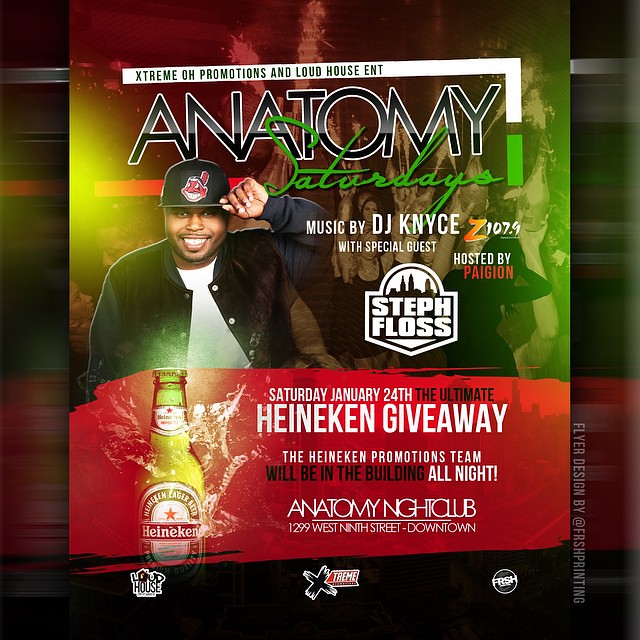This promotional poster for Anatomy Nightclub is a visually striking advertisement featuring a layered photographic and graphic design composition. The poster is rectangular and horizontally aligned, with a darker, illegible background creating a sense of depth. 

The top of the poster features a white banner with the text "Extreme Promotions and Loud House ENT". Below it, in large outlined letters, "ANATOMY" is prominently displayed, with the word "Saturdays" in a bold, green cursive script overlaid at the lower right.

An African-American male in his late 20s is centrally placed beneath the headline. He is smiling, making eye contact, dressed in a black jacket over a white shirt, and a black baseball cap featuring a red cartoon Native American logo. His left arm is raised, holding the cap's visor. To his right, in white text, it states, "Music by DJ K-NYCE" with "Special Guest" beneath, followed by a prominently displayed "Z107.9" and "Hosted by Paijian."

The bottom third of the poster features a vivid red, painted background with a green Heineken bottle on the left, surrounded by splashes of liquid. Adjacent text in white reads, "Saturday, January 24th - The Ultimate Heineken Giveaway - The Heineken promotions team will be on the dance floor all night." Below, in large white letters, the address "Anatomy Nightclub, 1299 West 9th Street, downtown" is provided.

Logos for Loud House, Extreme, and Fresh Printing are positioned towards the bottom, enhancing the event's branding and partnership promotions. This colorful and detailed poster not only captures the essence of the upcoming event but also highlights key details and participatory elements, ensuring potential attendees are well-informed.